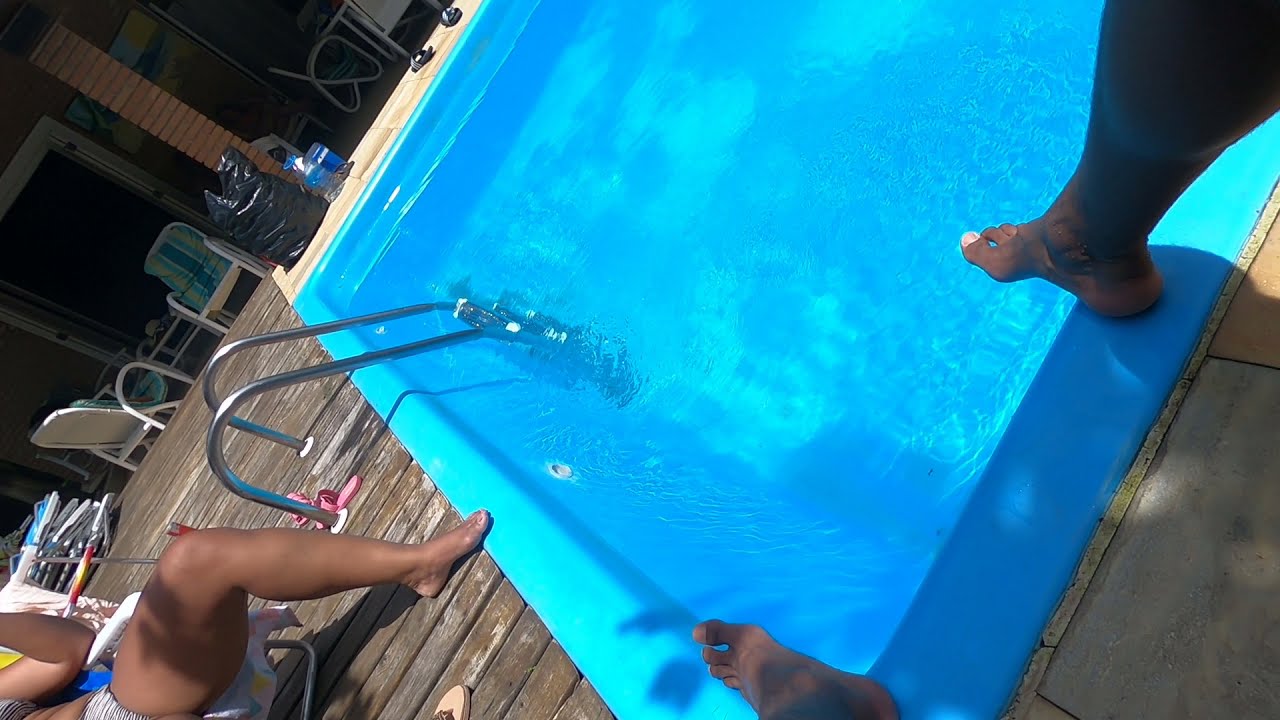This photograph captures a vibrant swimming pool setting from the perspective of a person dangling their legs over the water. The image is slightly tilted to the left, emphasizing a bright, clear blue pool that occupies part of the frame. The pool's edge features silver handrails leading into the water, and the surrounding area includes a brown wooden deck. On this deck, to the left of the image, is another person partially visible, seated on a lawn chair, with just their hands and legs showing. The scene reveals a sunny day with a well-maintained pool area. Further away, there are empty lounge chairs with blue and green cushions on white frames, and a reddish brick pillar. Below the pillar, a black trash bag and some clear bottles are scattered on the ground, adding minor details to this serene yet lived-in poolside environment.